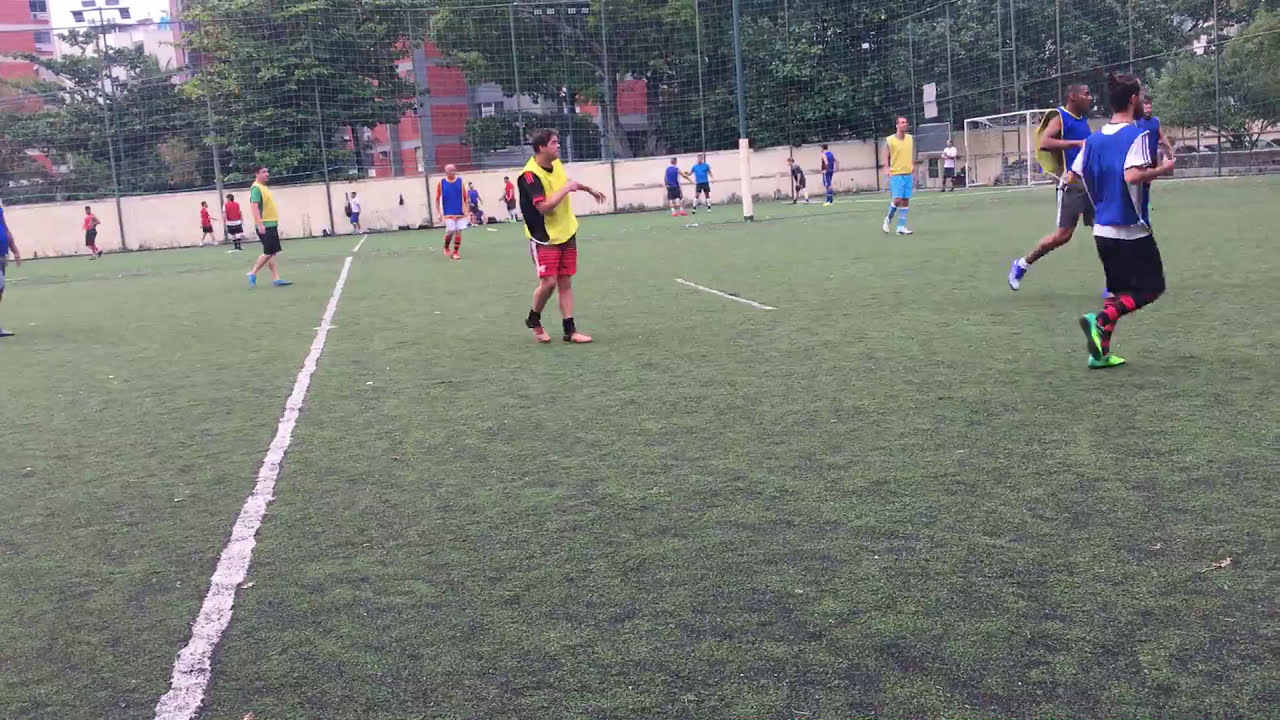This outdoor daytime photograph captures an ongoing soccer match on a lush green field with thin, sparse grass, highlighted by a central white line painted from the lower left to the midpoint of the image. The players, centered in the frame, are divided into two teams distinguished by their vibrant gear - one team in yellow shirts and red shorts, the other in blue shirts and black shorts. They are actively engaged in the game, their movements and varied ethnicities adding dynamic energy to the scene. Surrounding the field is a tall chain-link fence, and beyond it, a cream-colored wall stretches alongside trees and multi-story red buildings, creating a juxtaposed backdrop. The setting, vividly colored with tones of green, white, yellow, red, blue, tan, and black, suggests a lively day of outdoor sport, emphasized by the clear view of the goalposts and the encompassing net around the soccer field.